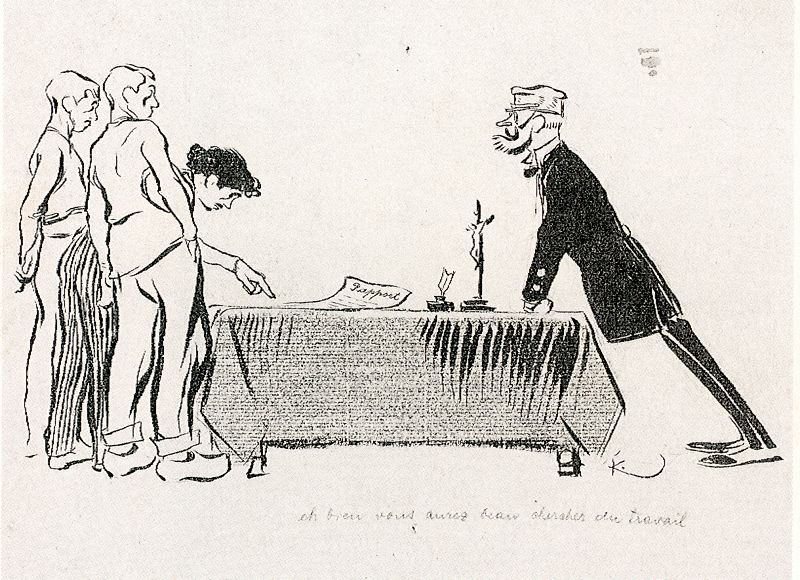In this detailed black and white cartoon drawing, four individuals are gathered around a table, likely in the midst of a negotiation or discussion. On the left side of the table, two individuals are standing beside a central figure who is bending forward. This central figure, characterized by black hair and wearing a dress with black and white stripes, is pointing at a piece of paper on the table, possibly a contract or proposal.

Standing opposite them, on the right side of the table, is a man dressed in black attire, including a coat, trousers, and shoes. He has a beard and appears to be wearing glasses. This man is leaning over the table at a sharp angle, with his knuckles firmly planted on the table as he glares at the others. His feet are set back from the table, giving him a menacing posture. Tucked under the arm of one of the standing individuals is a cap.

The table itself is draped with a cloth, obscuring its legs, and features several items: an inkwell with a feather pen, the possibly labeled paper, and a small cross with an image of Jesus Christ. The overall scene suggests tension and the importance of the document in the negotiation process. At the bottom of the image, there is some unclear text, adding to the comic strip style of the illustration.